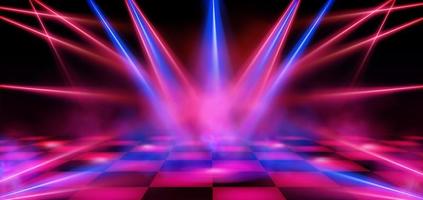The image captures a nostalgic disco dance floor with a distinct black and pink checkered tile pattern. Neon lights in vibrant shades of blue, red, and pink illuminate the scene, with blue lights predominantly shining from the bottom corners and red lights streaming from upper sections of the image. These neon beams create a laser light effect, reminiscent of the disco era's energetic ambiance. The black background complements the checkered tiles, adding depth and contrast. A subtle fog hovers just above the floor, enhancing the image's retro vibe and creating a captivating play of light and shadow.